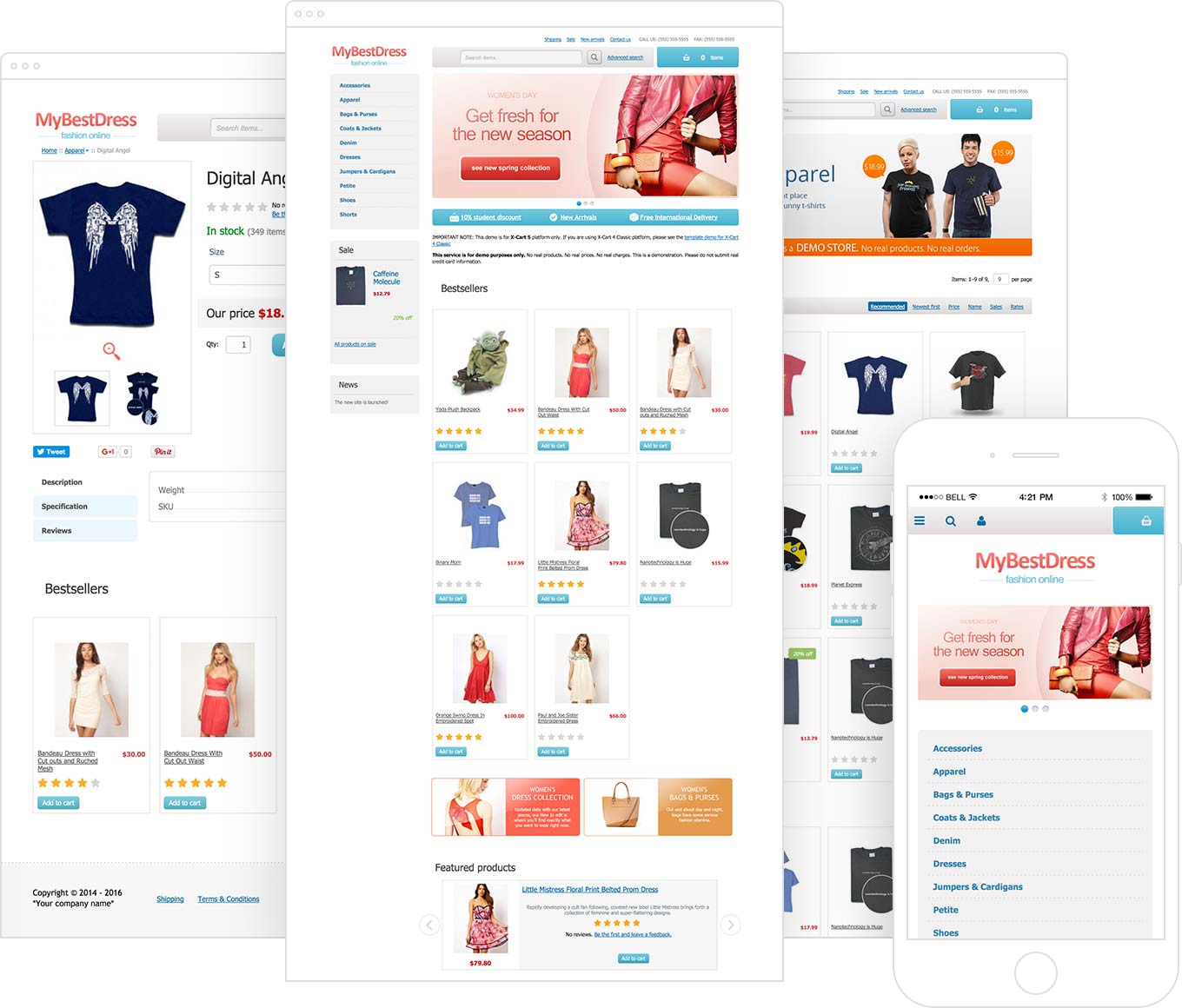This image features four smartphone screens displayed against a white background. 

1. The first phone screen shows a shopping app with various UI elements. At the top, there are small purple lines followed by the text "My Best Dress" in pink. Below this, there's a purple search bar. An image of a blue t-shirt with angel wings is situated near a blue Twitter icon, accompanied by pricing details on the right. Towards the bottom, there's a section titled "Bestsellers" showcasing a sleep shirt and a two-piece outfit, each with blue buttons beneath them.

2. The second phone screen also displays "My Best Dress" at the top with a search bar nearby. It features a blue box to the left listing different items, another blue box indicating "Sale," and a third blue box at the right. A large pink box on the right side displays an image of a girl in a pink outfit with the text "Get Fresh for the New Season" above a red button. Below this, another blue box with white text is visible. The "Bestsellers" section showcases eight different items, followed by two larger images and a "Featured Products" section with a dress rated five stars and a blue button beneath it.

3. The third phone screen showcases an "Apparel" section at the top with an image of two men in short-sleeve shirts. Below this, an orange box reads "Demo Store." Several t-shirts are listed with their prices and a blue "Buy" button, followed by more shirt listings underneath.

4. The fourth phone screen displays three dots at the top and "My Best Dress" text with a pink picture below it. This is followed by a blue box featuring various items. At the bottom, the screen features three dots, with the first dot in blue indicating the current page, displayed over a large white circle.

Overall, the image visually represents a detailed interface of a shopping app as displayed on four different mobile screens.